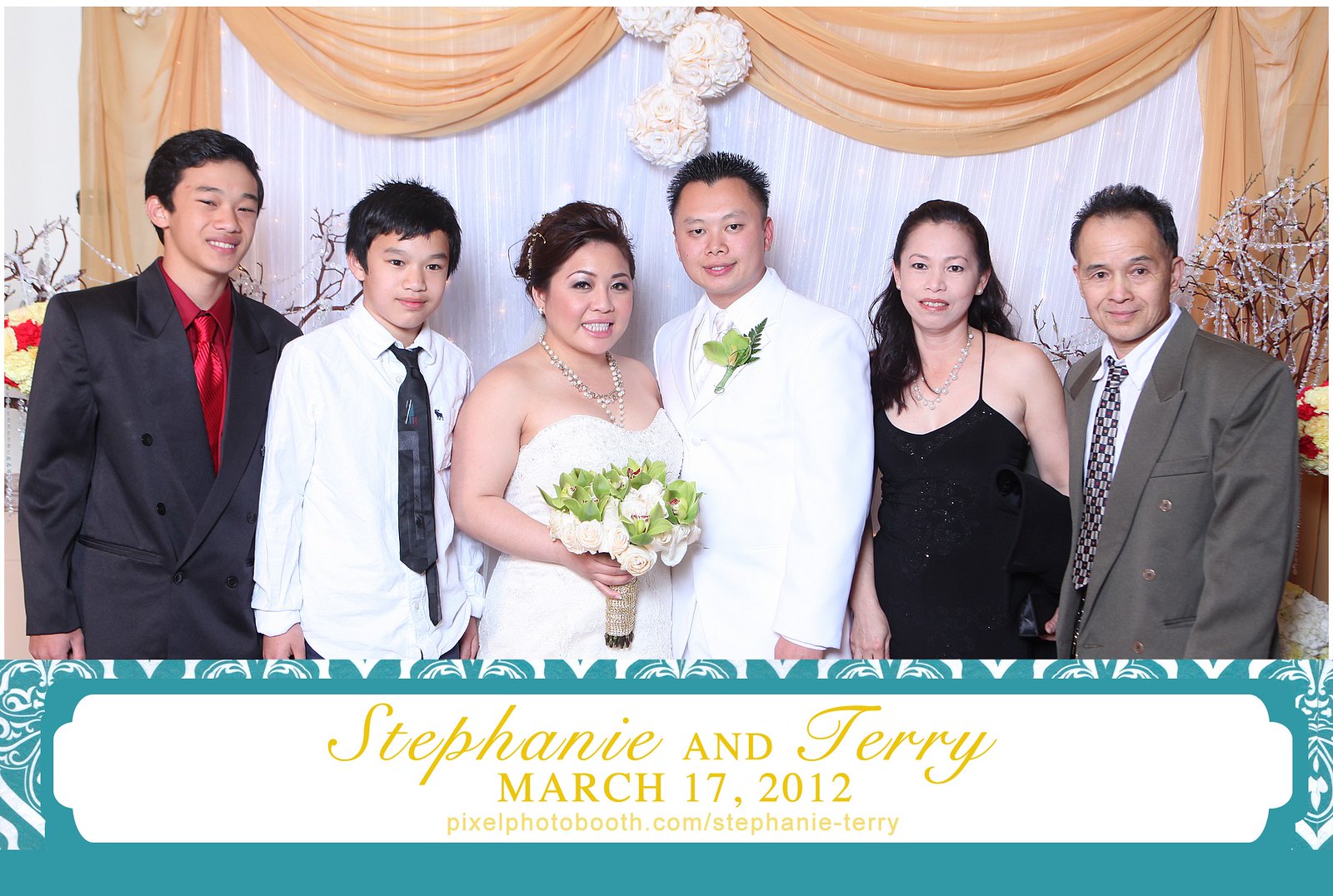This detailed wedding photograph captures a celebratory moment with six people of Asian descent, all standing in a horizontal row. At the center are the bride and groom, prominently positioned in radiant white attire. The groom adorns his suit with a green floral lapel decoration, while the bride holds a stunning bouquet of green and white flowers. To the bride’s right stands a young boy in a long-sleeve white dress shirt, untucked, paired with a dark tie. 

On the far left of the image, a man dons a gray suit, complemented by a red dress shirt and red tie. Next to the groom, on the left, is a woman elegantly dressed in a black strapless gown. Completing the group, another man in a gray suit with a white dress shirt and a square-patterned tie stands next to her. The backdrop showcases a sheer white curtain with beige sheer accents, adorned with puffy white bow-like decorations in the center. 

At the bottom of the photograph, a turquoise banner displays “Stephanie and Terry, March 17, 2012,” with the inscription “pixelphotobooth.com/stephanie-tery” in yellow letters. The predominant colors in the scene are white, gray, and shades of yellow and red, adding to the festive and elegant atmosphere of this cherished moment.